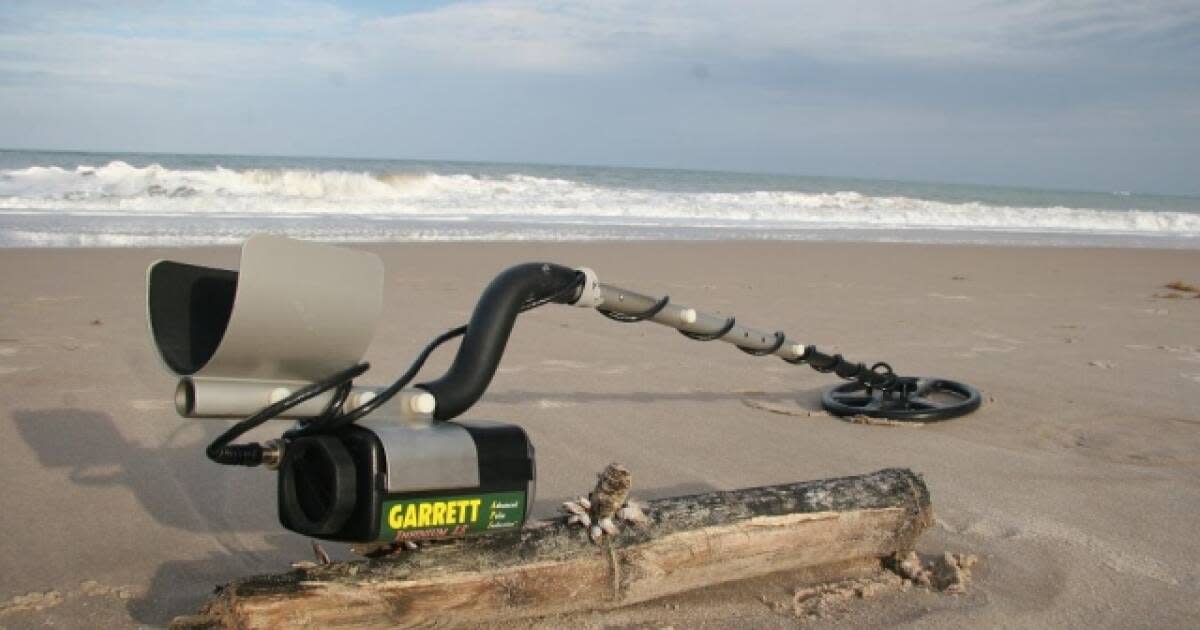This photograph captures a detailed scene on a beach during the daytime. In the foreground, the wet, brown sandy surface is prominently visible. A small, sand-covered wooden log, possibly driftwood, lies diagonally from the lower left to the upper right, adorned with seashells, suggesting either natural decoration or marine life growth. Resting against this log is a metal detector, identifiable by its silver and black structure. The brand, Garrett, is clearly marked in yellow on a green tag attached to the device's battery pack. The metal detector has a gray pole, with a black, curved section providing a supportive arm cuff. A black wire coils around the pole, leading to a circular detection pad resembling a steering wheel at the end. In the background, a narrow band of bluish-green ocean waves, capped with foam, rolls onto the shore. The horizon meets a grayish-blue sky filled with scattered gray clouds, completing the scenic beach vista.